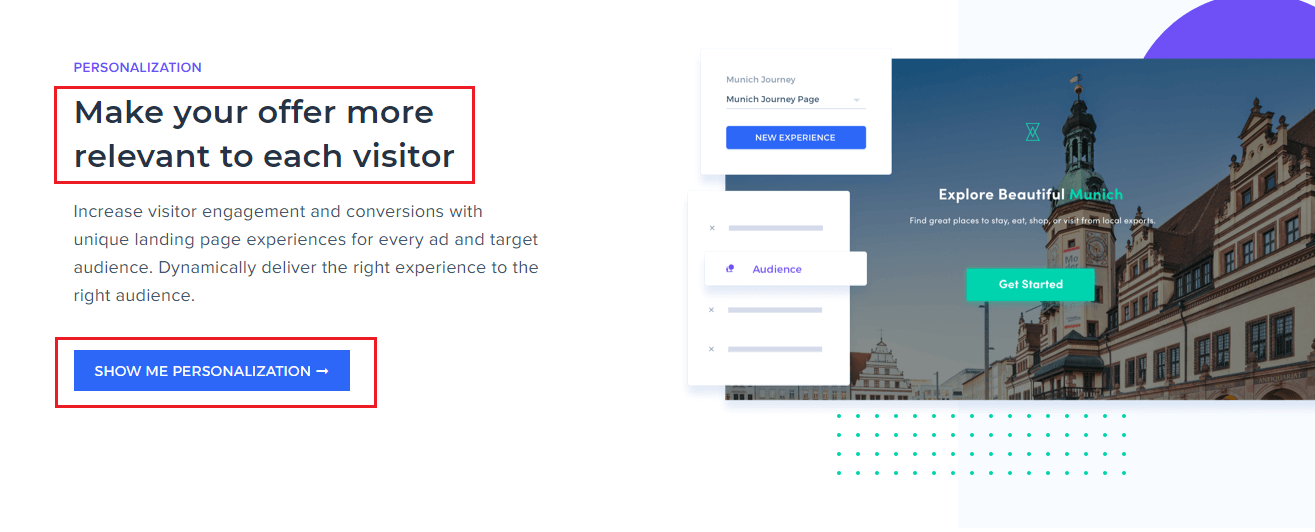The image is a rectangular screenshot of a webpage with a focused section about personalization. The top left corner features the word "Personalization" in a vibrant purple font. Below this, a block of text is enclosed within a red border. The text within the box reads: "Make your offer more relevant to each visitor." Further down, additional text states: "Increase visitor engagement and conversions. With unique landing page experience for every ad and target audience. Dynamically deliver the right experience to the right audience."

A prominent button is situated below the text, framed with a red border and inscribed with the phrase "Show me personalization."

On the right side of the image, there is a background featuring a multi-story white building with numerous windows. Behind this building, the sky is visible, adding a picturesque element to the composition.